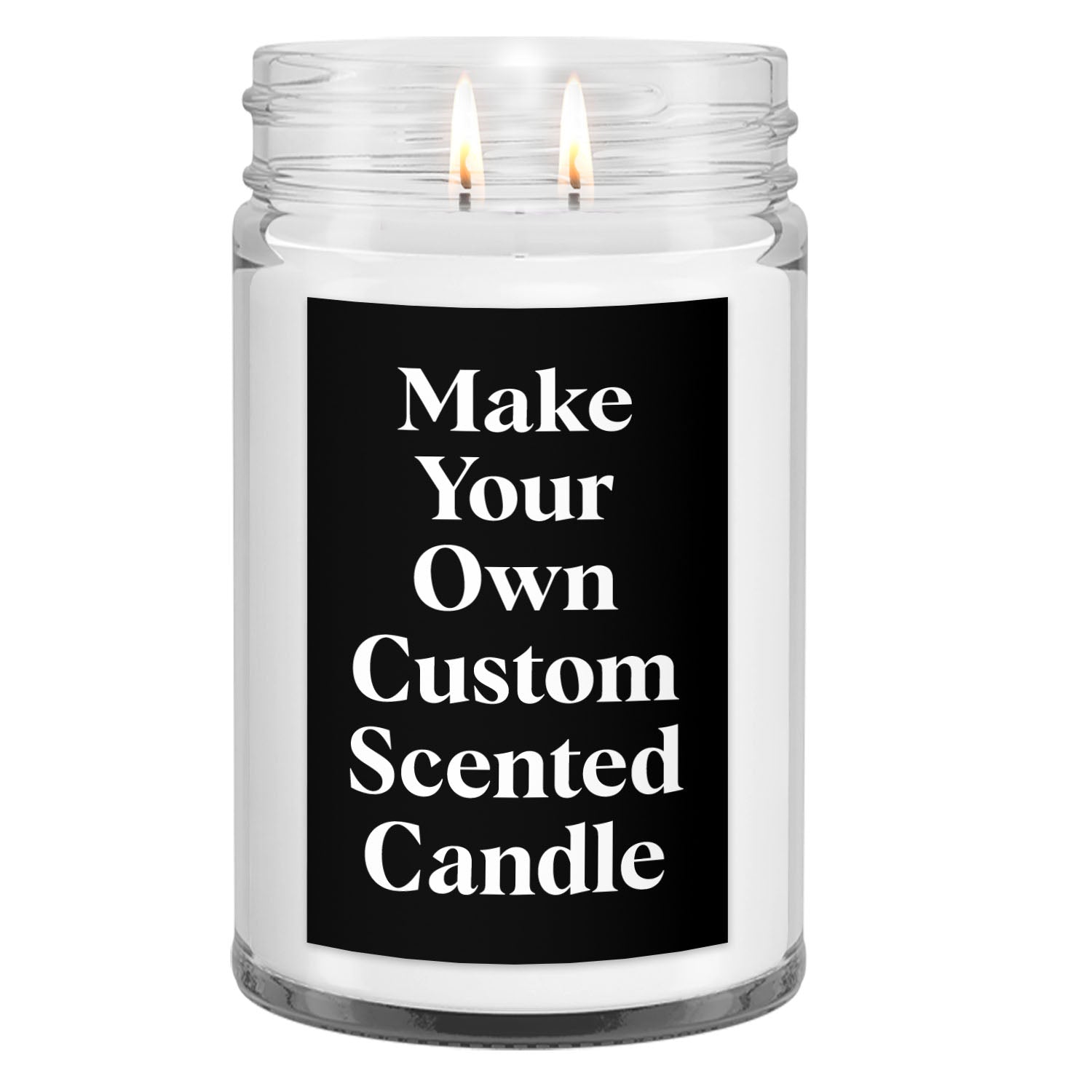The image depicts a close-up of a glass jar candle with two lit wicks, casting warm, flickering flames. The candle's wax is white and its container is a clear, cylindrical jar that transitions seamlessly into a threaded neck suitable for a screw-on lid. The flames are contained just below the jar's mouth, adding a cozy glow without extending above the jar’s edge. Front and center on the jar is a black rectangular label with white text displaying "Make Your Own Custom Scented Candle," indicating it's an advertisement for customizable candles. The background is entirely white and transparent, likely to emphasize the candle and its label, making it suitable as a display photo for a website or promotional material.